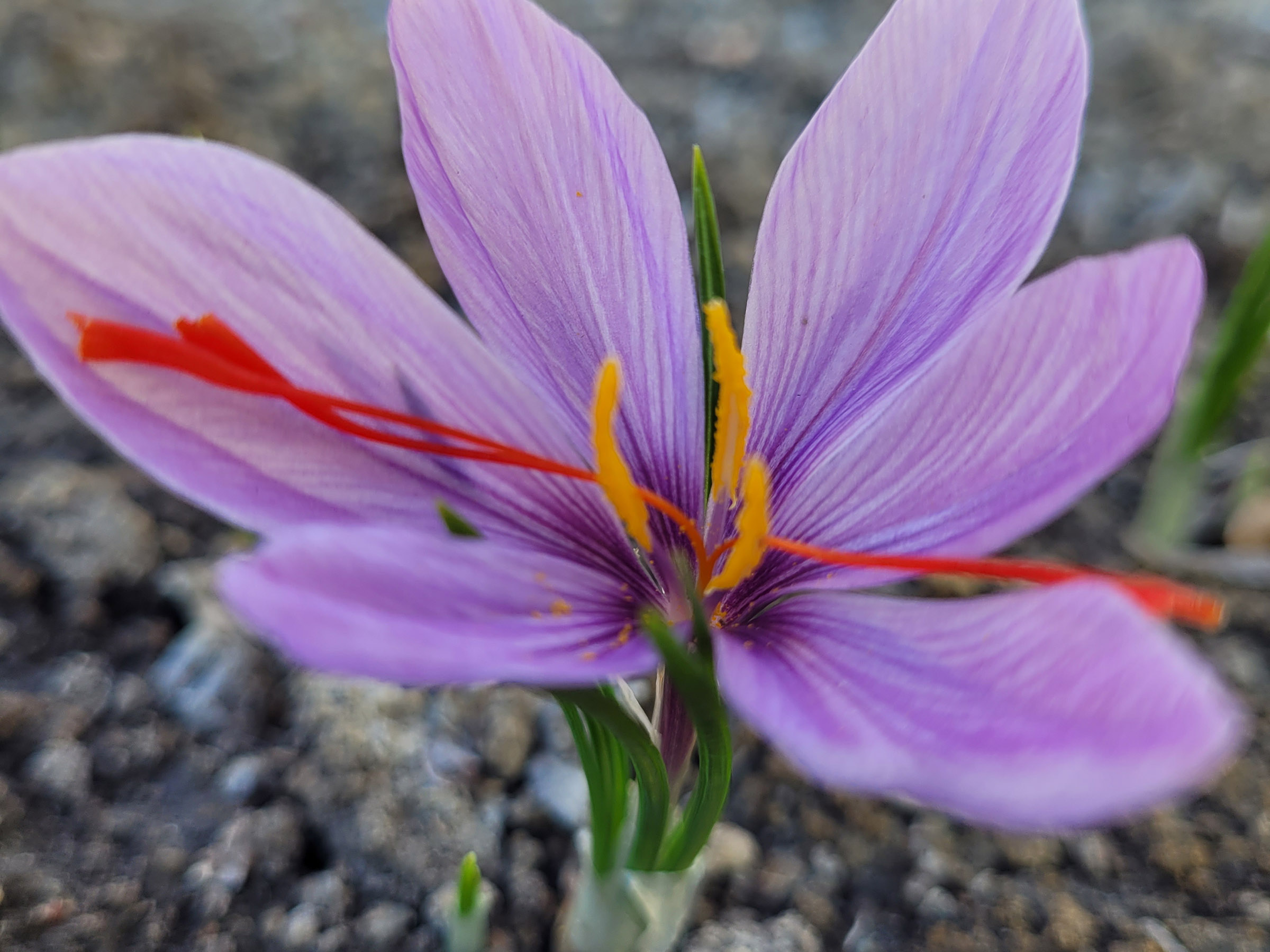This close-up image captures a striking purple flower with six elongated, curved petals, each displaying intricate, thin, deep purple veins. Emerging from the center, three upright yellow stamens coated in vibrant pollen contrast with three peculiar, vivid red filaments that extend outward horizontally like strings. The green stems of the flower peek through and support it from below, fading into a softly focused, rocky, grayish background that adds texture without drawing attention away from the flower's intricate details.